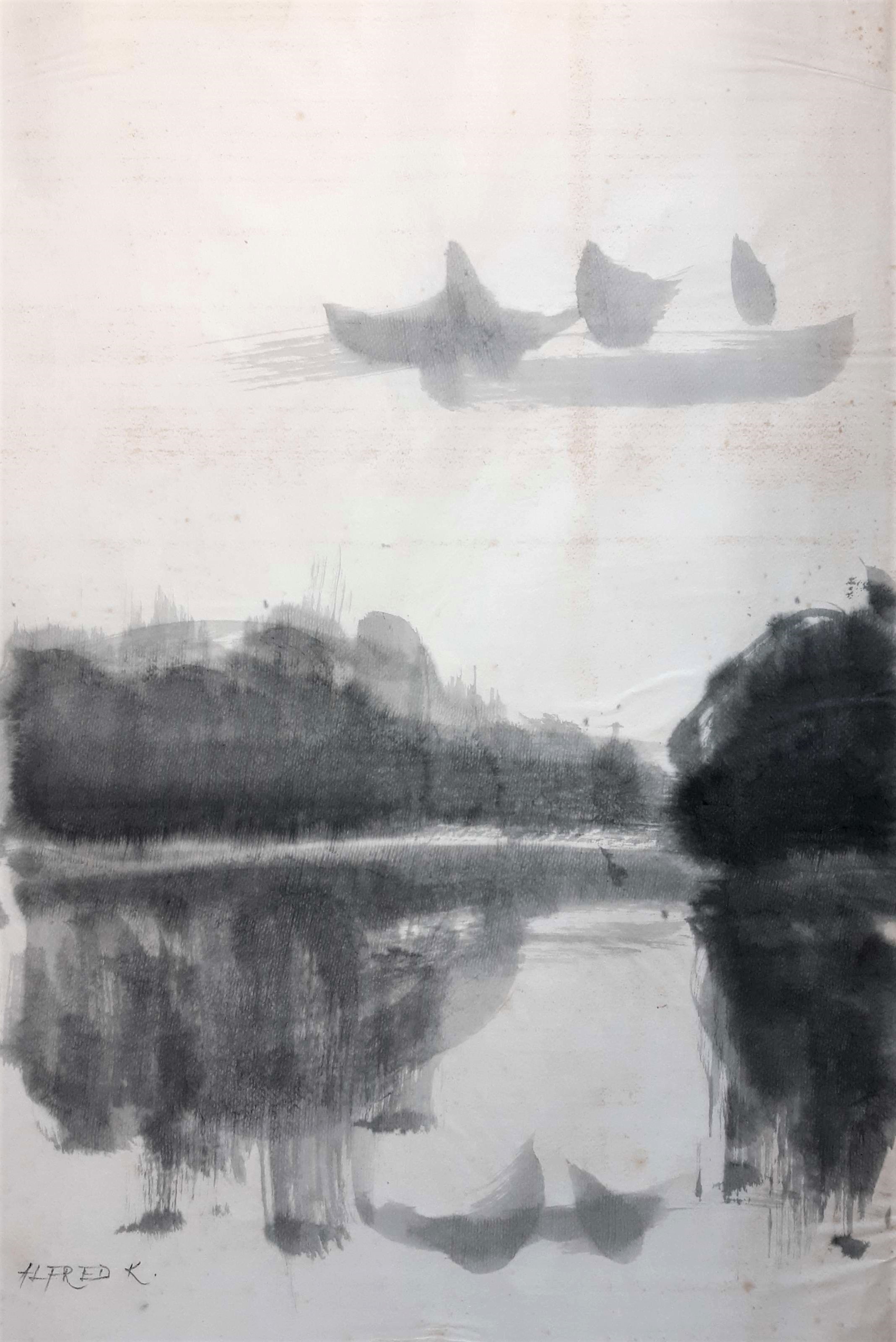This abstract black-and-white artwork appears to be a watercolor or charcoal painting, depicting a serene lake scene. The composition features amorphous shapes, possibly representing the surrounding forest or mountains, which are dark and reflect off the lake's surface. On the lake, a small bird, perhaps a goose or duck, is visible. The sky contains several cloud-like blobs, also reflected in the water, alongside a surreal image of a boat floating in the sky with birds in or around it. The overall color palette consists of shades of white, gray, and black. Additionally, the bottom left corner of the painting bears the text "Alfred K," likely the signature of the artist.